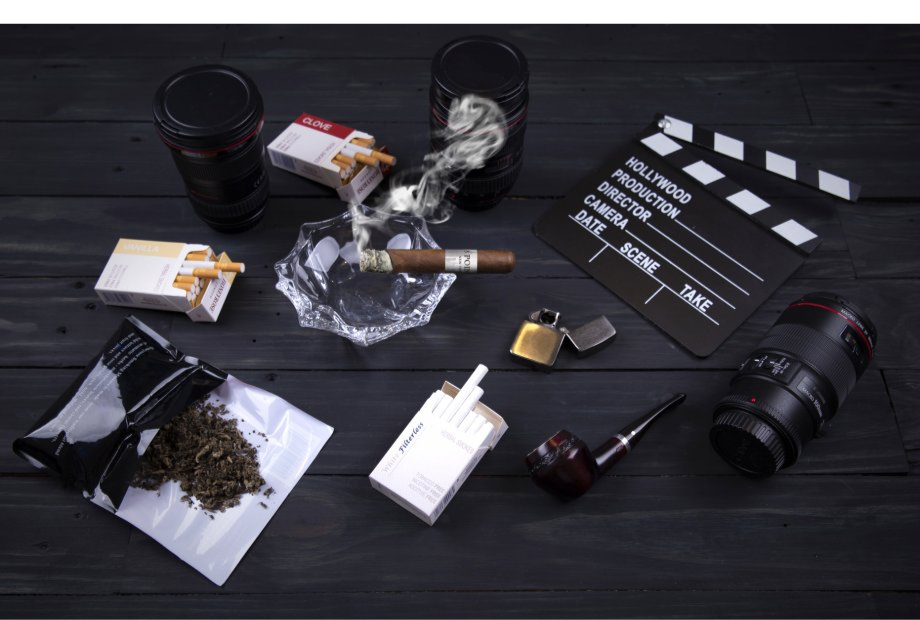The photograph showcases a variety of items seemingly strewn on a black wooden surface, possibly as movie props. Central to the image is a Hollywood clapperboard in classic black and white, with inscriptions that read "Hollywood Production Director Camera Date Scene Take." Surrounding it are three packs of cigarettes, each with a couple of cigarettes protruding from their tops. Directly below the clapperboard is a camera lens, while another lens is positioned to its right, and a third to the far left. Notably, an open pouch spilling loose tobacco sits to the left of the clapperboard. Adjacent to this is a metallic, golden Zippo-style lighter. Also present is a tobacco pipe situated left of the clapperboard. Tucked beneath the pouch is a crystal ashtray, housing a lit cigar with tendrils of smoke rising from it. Additionally, the setup includes a pair of black thermal glasses, each with lids, and a small lock placed among the items. The arrangement of these items suggests a meticulously curated collection of props, focusing heavily on smoking-related items and cinematic apparatus.